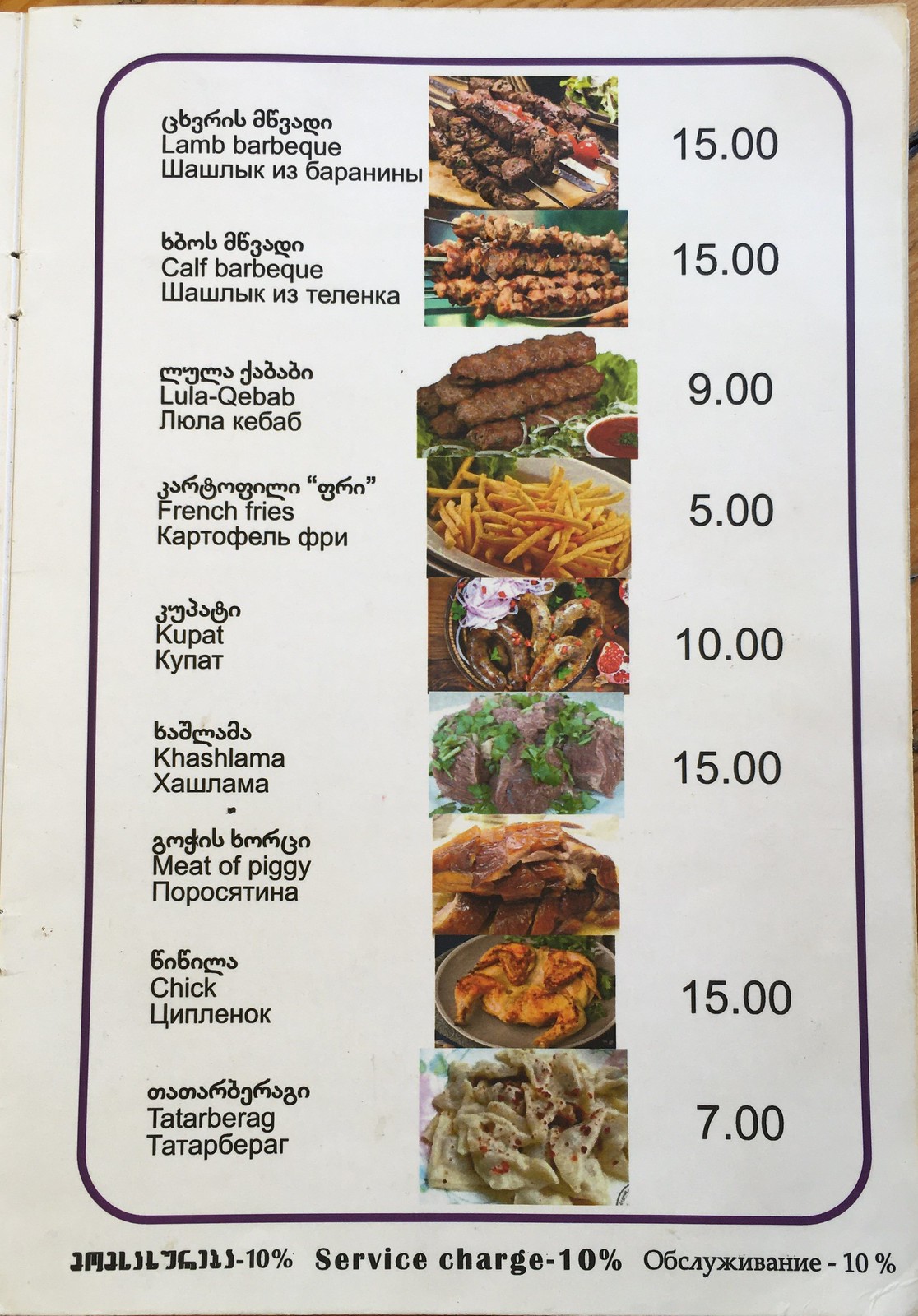This is a detailed photograph of a menu page. The menu has a clean, white background with a black square featuring rounded corners, encompassing the listed items. The text on the menu is in black, with item names and prices clearly separated by corresponding food images. From top to bottom, the menu items include lamb barbecue, calf barbecue, lula kebab, French fries, cupot, kashama, pork meat, chicken, and tater barak. The text is organized with English translations centrally positioned, while the top portion appears to be in Arabic, and the bottom section in Cyrillic script, possibly Greek or another language using the Cyrillic alphabet. At the very bottom of the menu, a note states a 10% service charge, which is written in all three languages for clarity.